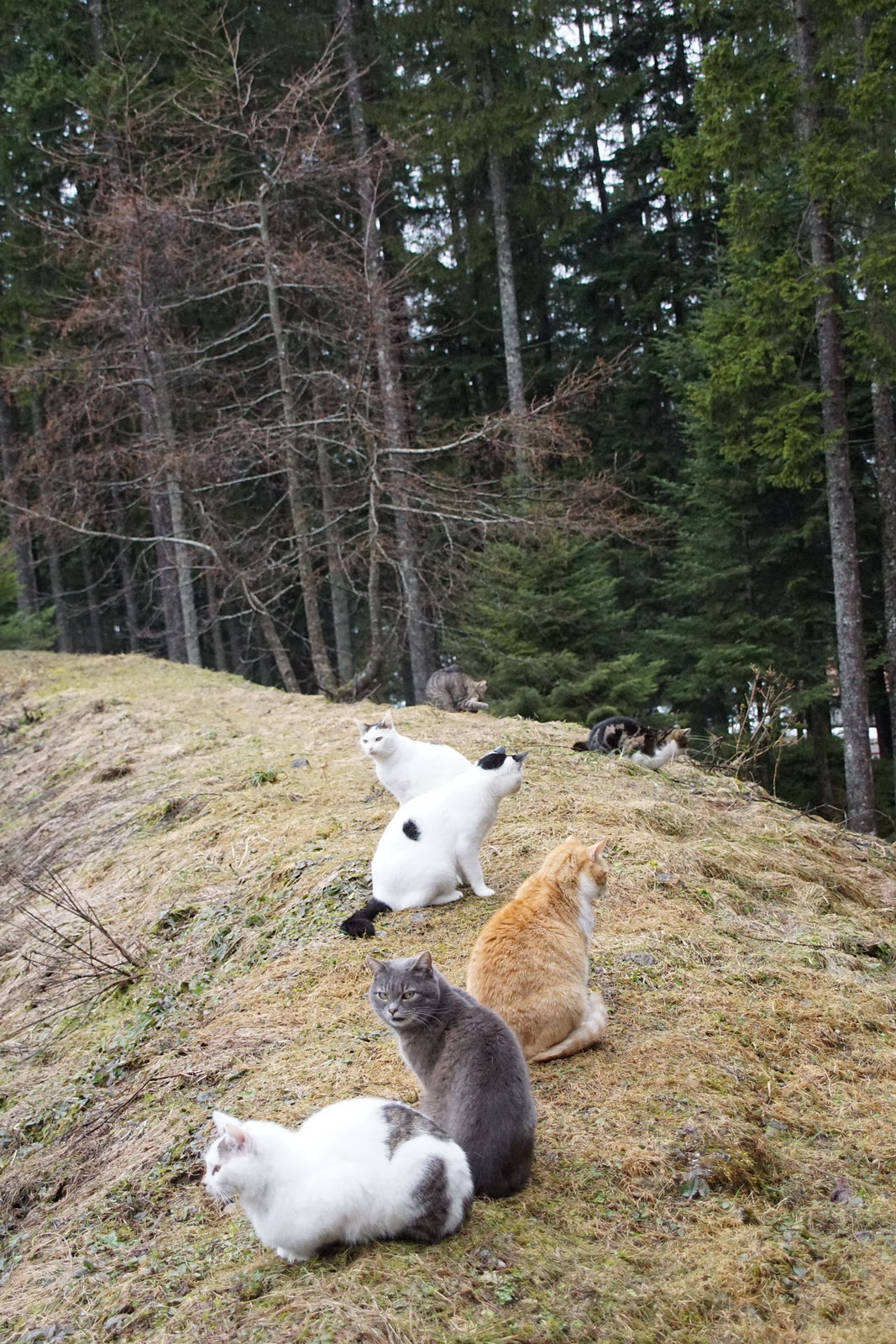This outdoor photograph captures a picturesque scene of a small, grassy hill, browned and patchy with some surviving green spots. Atop the hill, a charming group of cats commandeers the focal point. The nearest feline, a white cat with gray stripes on its back haunches, lies comfortably at the forefront. Next to it, a gray cat sits gazing behind. Beside the gray cat is an orange cat whose attention is fixed toward the distant trees. Nearby, another white cat with dark ears, a prominent black spot on its back, and a black tail also looks at the forested background. Among them, an additional white cat with subtle black markings on its head faces the camera. The background unveils a picturesque forest with a mix of bare, gray trees and vibrant evergreens. Further in the distance, a variety of other cats add to the visual symphony: a gray tabby, a calico with a white chest, and a cat patterned in black and orange. The entirety of the hill exhibits a weathered appearance, suggestive of grass that has been flattened by snow, awaiting the renewal of spring.